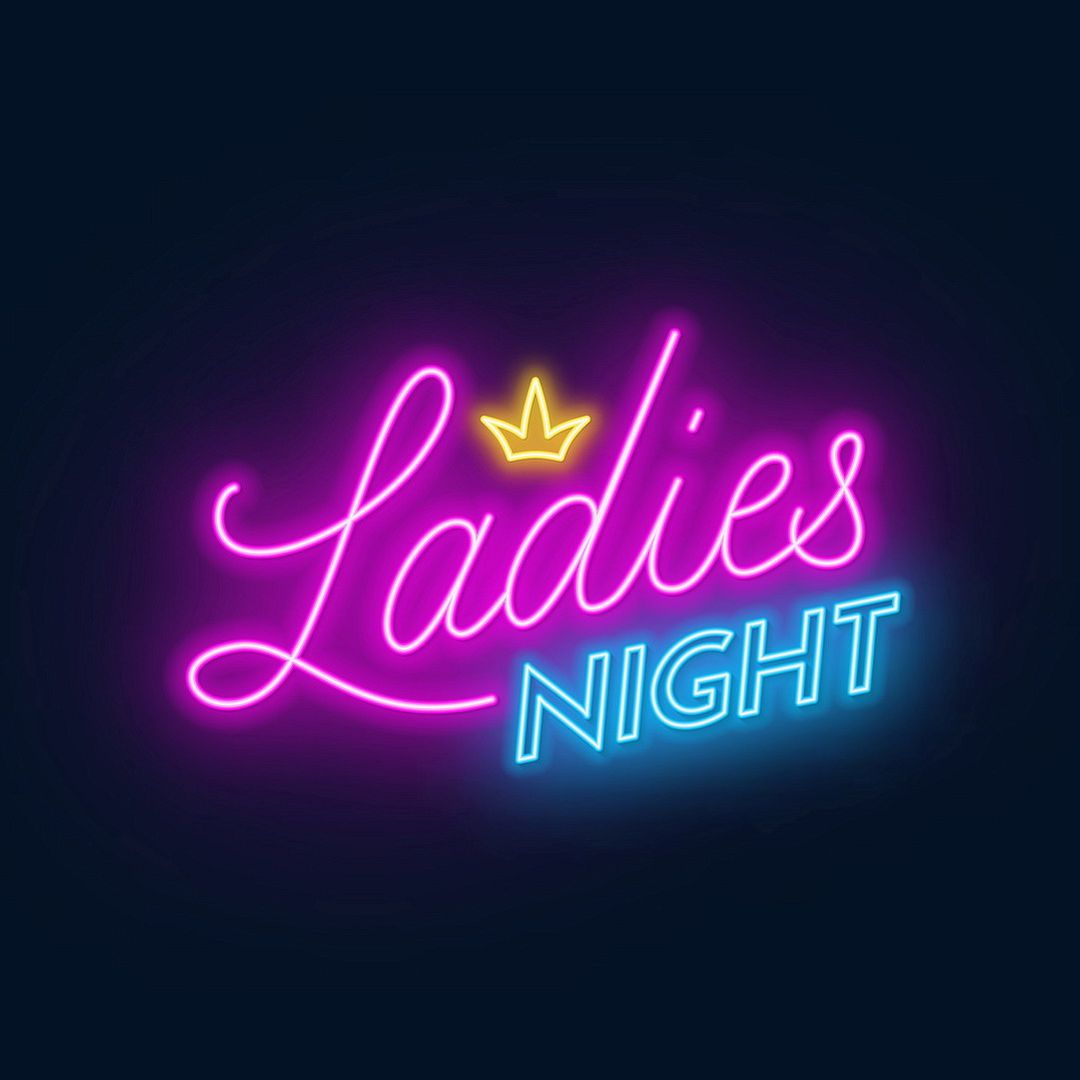In this image, a vibrant neon sign stands out against a black background. The centerpiece of the sign is the phrase "Ladies Night," illuminated in striking neon colors. "Ladies" is written in a cursive, handwritten style using a mix of light pink and purplish tones, and it stretches diagonally from the left to the right. Above the "Ladies," positioned over the letters "A" and "D," there is a yellow-gold neon crown featuring three points—two shorter ones on the sides and a taller one in the center. The word "Night" is displayed in a bold, uppercase font beneath "Ladies," beginning near the "D" and extending diagonally in lighter blue letters with a subtle darker blue background glow. The entire sign casts a vivid, eye-catching contrast against the dark backdrop, creating a lively and inviting atmosphere.